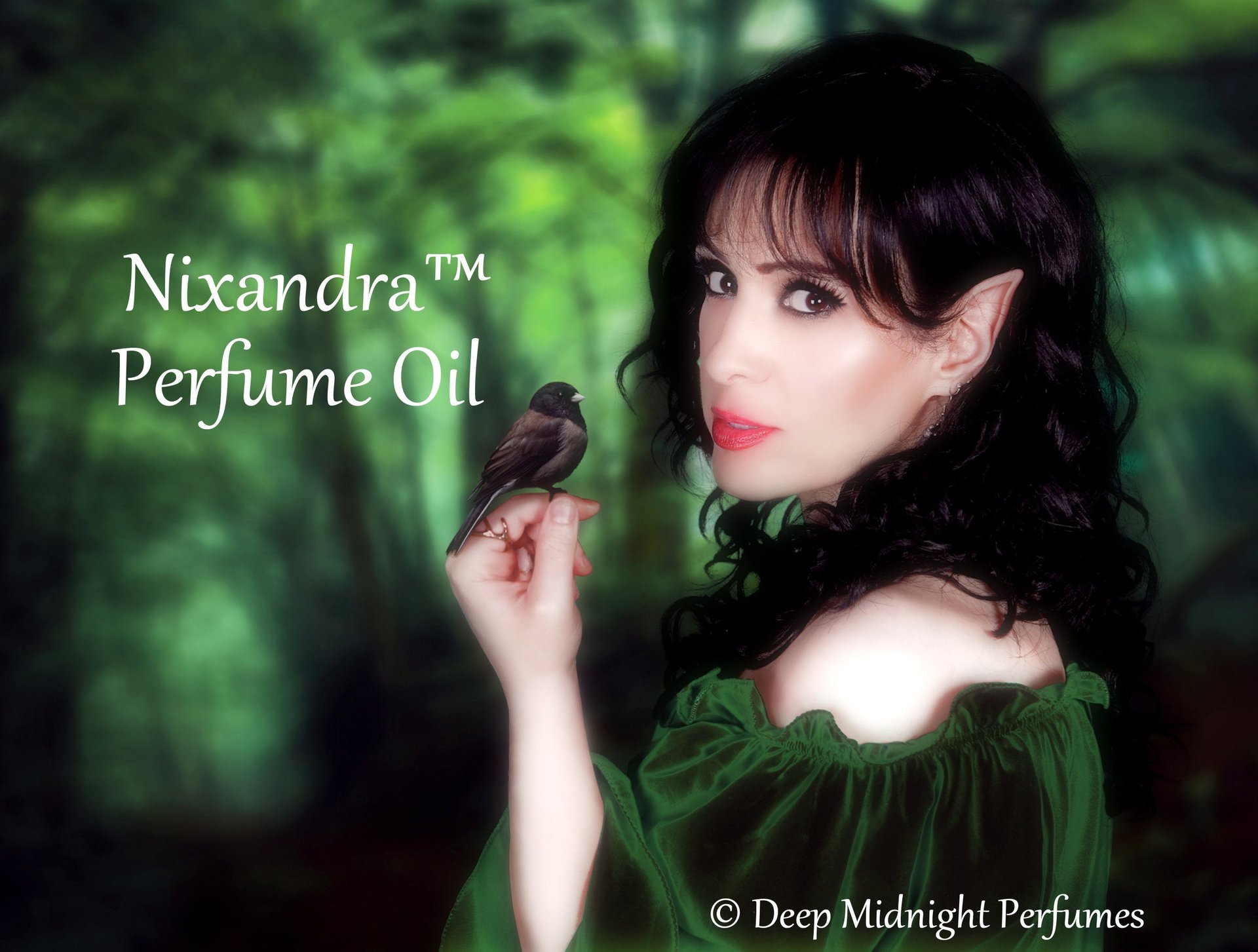The image features a white-skinned woman with black hair that cascades past her shoulders in loose waves and curls, settling around chest level. Her curly hair frames both sides of her face, with some strands falling in front and others behind her shoulders. Highlighting a fantasy theme, she has distinct elf-like pointy ears. She is wearing a green, velvet-like dress with ruffles, designed with an elastic band that leaves her shoulders exposed, revealing her skin. She has striking red lipstick and heavy mascara, making her eyes stand out as she gazes directly at the camera. Her body is angled to the left, with her left shoulder prominently visible, and her left hand is raised vertically, holding a small, dark, grayish-black bird with a yellow beak.

The background is a lush, vibrant green, evoking a sense of foliage, possibly comprising trees and bushes. Prominently displayed in the top right corner in white text is "Nixandra™ Perfume Oil." In the bottom right corner, right above her dress, the image has a copyright symbol followed by "Deep Midnight Perfumes." This detailed scene is part of an advertisement for Nixandra Perfume Oil, blending elements of nature and fantasy.